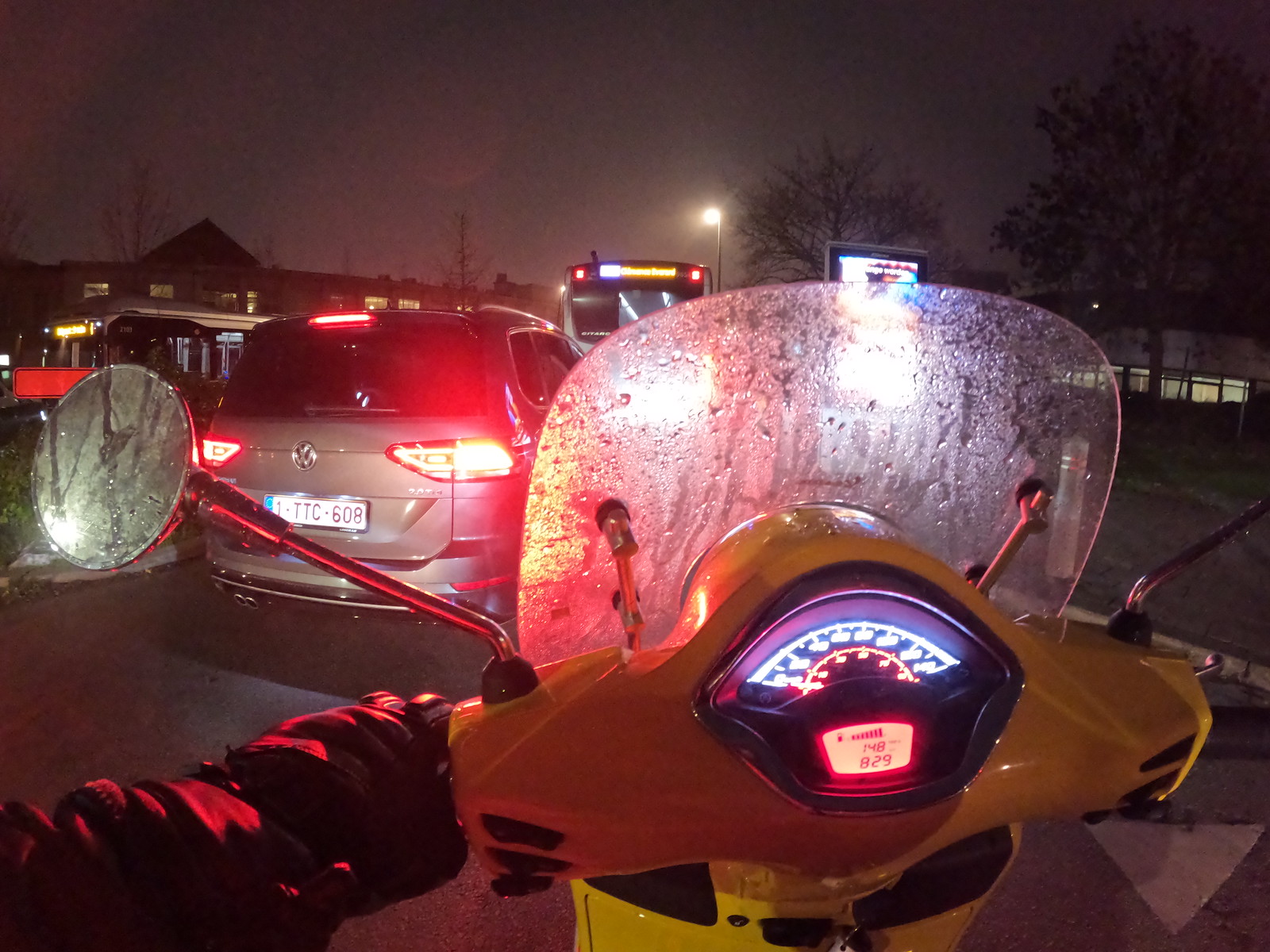The nighttime scene captures the perspective from a stationary motorcycle. The rider's hand, clad in a black glove and extending from a long black sleeve, grips the yellow handlebar of the motorcycle in the lower left corner of the image. A small windshield in front of the handlebars shows signs of condensation and rain. The blue-lit speedometer, displaying the number 829 in red, adds a distinct glow to the scene. To the left, the motorcycle's rearview mirror reflects the dark surroundings, while in the distance, the brake lights of a gray Volkswagen SUV are visible. Further ahead, a city bus with a neon-lit sign atop stands illuminated under a white streetlight against the dark gray sky. To the left side of the frame, the edge of a building with a peaked roof and some trees on the right add to the urban nightscape.